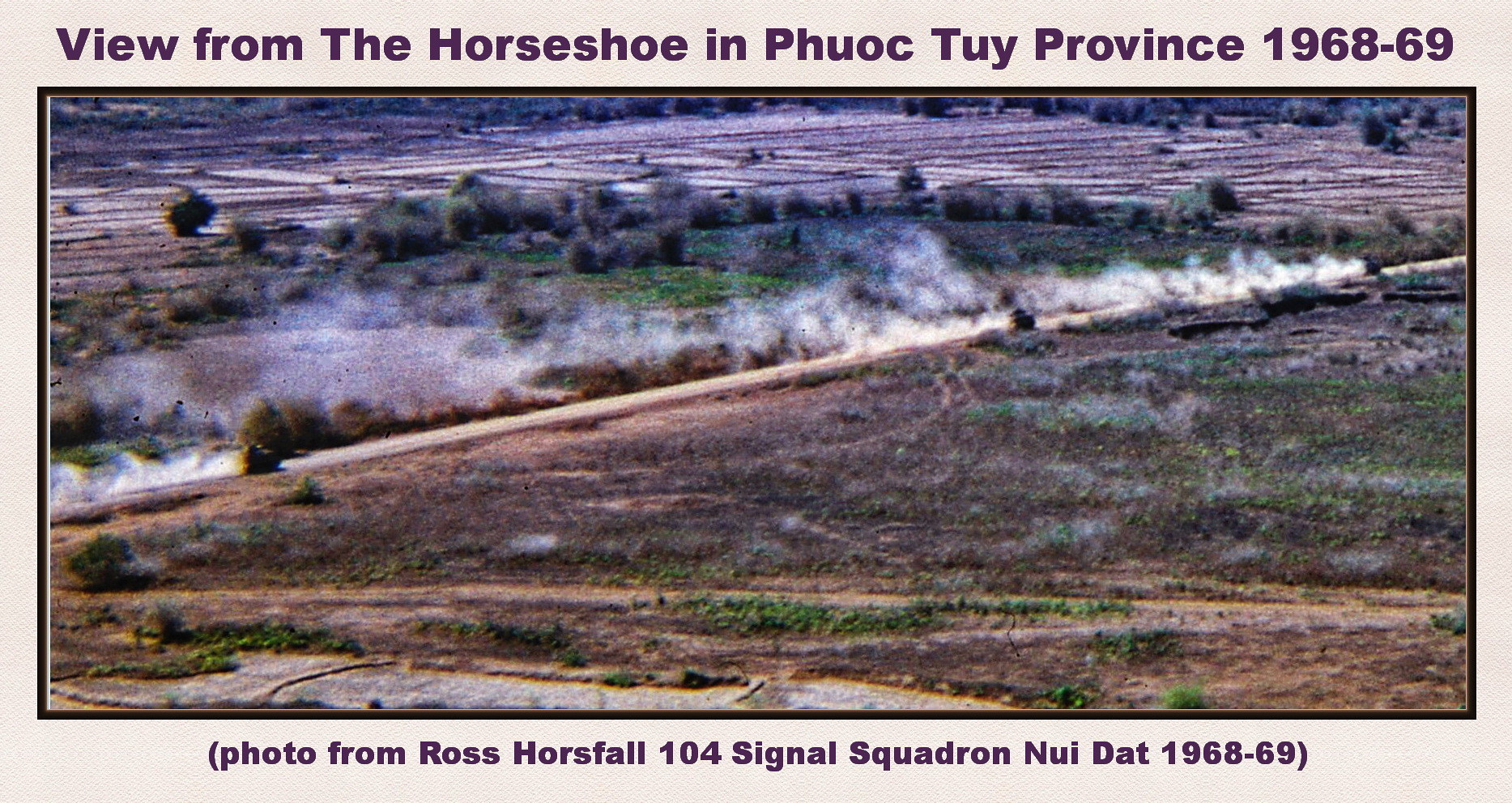The photograph, set against a white background with a light grayish-brown border, prominently features the title in bold purple text at the top: "View from the Horseshoe Inn, PHUOC TUY Province, 1968-69." The image, captured in landscape mode, reveals a misty, rocky terrain foreground leading into a barren field dotted with a few shrubs. The scene is dominated by a dirt road cutting diagonally from just below center left to the upper right corner, with three vehicles kicking up clouds of dust behind them. The muted colors in the photograph depict a field under a seemingly overcast sky, adding to the obscurity of the green and blue hues. At the bottom, in purple print, the footer reads: "(Photo from Ross Horsefall, 104th Signal Squadron, Nui Dat 1968-69)." This comprehensive view presents a snapshot of the historical landscape during the Vietnam War era, meticulously outlined by annotations that add context and detail.